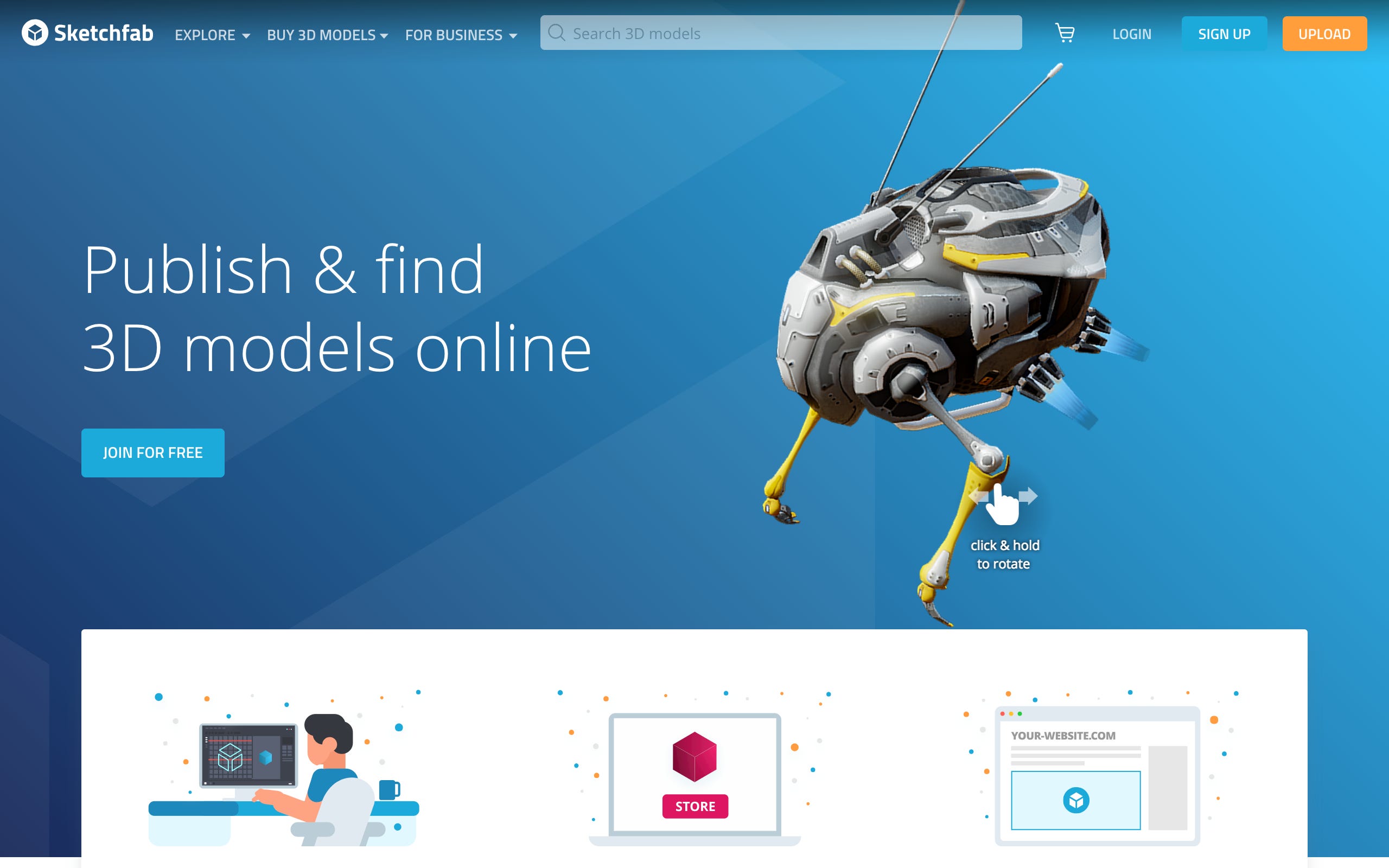The image showcases the web page of Sketchfab, an online platform dedicated to the exploration and purchase of 3D models, particularly for business purposes. The interface includes navigational links such as "Explore," "Store," "Login," "Sign Up," "Upload," and options to "Search for USA" or "Search 3D Models." The website encourages users to join for free, publish their 3D models online, and utilize features like clicking and holding to rotate the models. The platform, named Colossia, is visually branded with a color scheme of blue, white, yellow, and red.